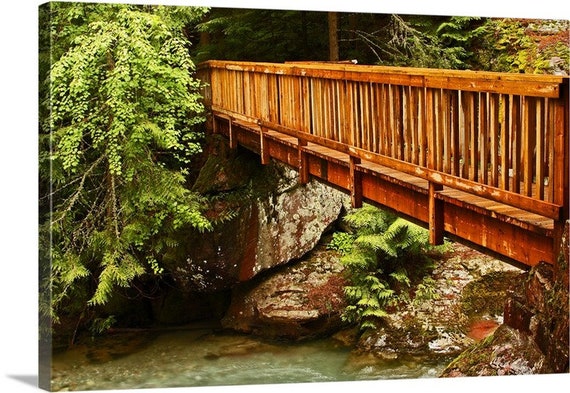The image is a highly detailed photograph of a wooden bridge, probably made from cedar or stained to a reddish hue, stretching across a clear, shallow stream in a mountain setting. The bridge, approximately 50 feet long, spans a rocky ravine surrounded by lush greenery, including mountain ferns, firs, and other evergreens. Large rocks, some as big as 10 to 20 feet in height and width, are scattered adjacent to the stream, adding to the rugged, natural beauty of the scene. The photograph captures the essence of a picturesque national park, exuding a sense of tranquility perfect for a hiking trail. The image itself is presented on a thick canvas, around an inch deep, akin to a wrapped photograph or a mounted piece of art that one might hang on a wall, enhancing the visual appeal with a three-dimensional effect.